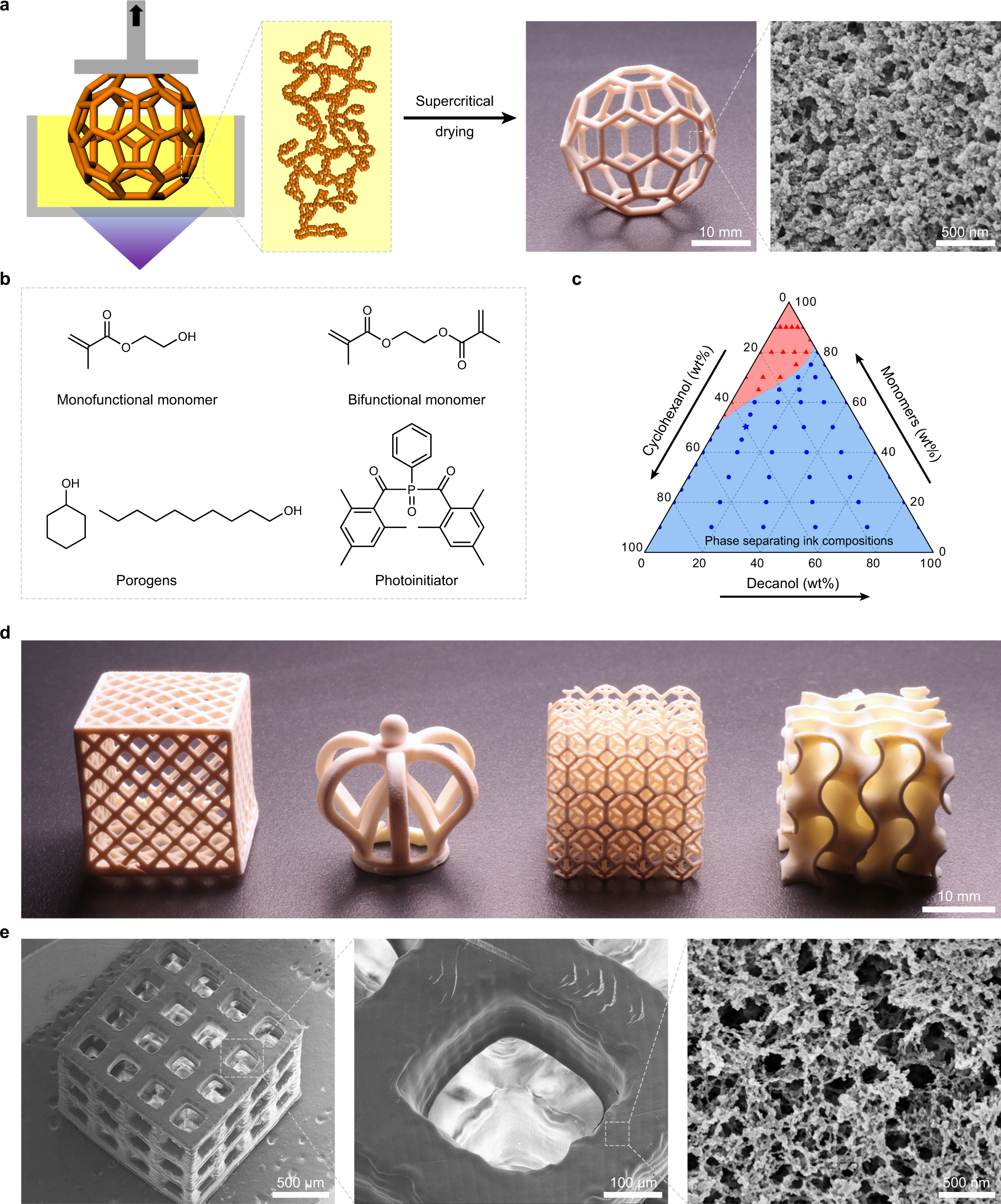This is a detailed and comprehensive informational set of images, likely from a structural chemistry or medical textbook, organized into five sections labeled A, B, C, D, and E. At the top left of section A, there is a spherical organic compound connected to another similar spherical drawing to the right. Directly below this in section A, line notations and descriptions of monofunctional monomers, bifunctional monomers, pathogens, and photoinhalators are featured. Section B presents simple molecular structures and drawings, including labels such as supercritical drying, further delineating different molecular forms. In section C, there's a pyramid illustrating measurements of decanol monomers and cyclohexanol. Section D showcases complex representations of molecules, which appear to be sculptural forms, possibly created with a polymer mold, resembling 3D printed structures. Finally, section E at the bottom contains three microscopic images, providing a black and white, zoomed-in view of the molecules. Each section builds on the previous, transitioning from simple diagrams to more complex and detailed forms, offering a richly layered visualization of the discussed chemical entities and structures.